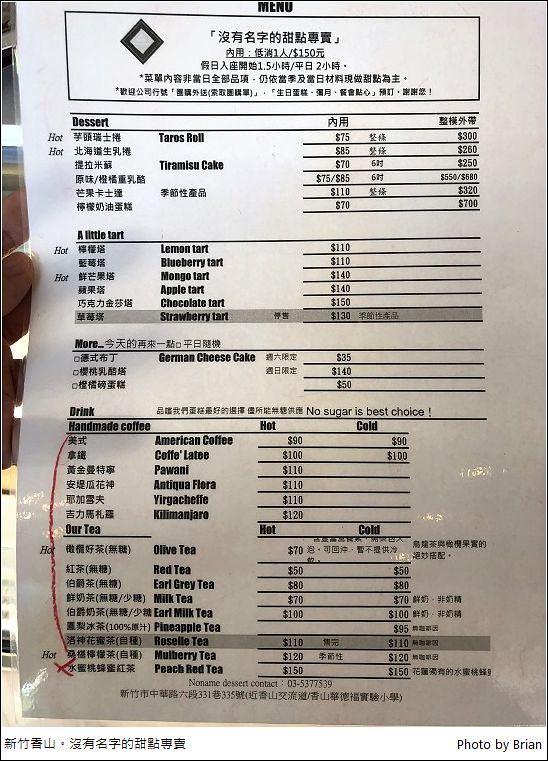This photograph showcases a menu from a country where English is not the primary language, featuring a mix of characters that could be Chinese, Korean, or Japanese. On the left edge of the image, a hand is holding up the menu. In the bottom-right corner, "Photo by Brian" is written, while the bottom-left features more oriental characters.

At the very top, the word "MENU" is written in block capital letters, partially cut off but still legible. Below it, a rectangular outline encloses a diamond logo and text in the native language. The menu is divided into different sections, each listing items in the original language alongside English translations and prices on the right.

In the "Dessert" section, there are six items listed. Two items are translated: "Taro Roll" and "Tiramisu Cake," with prices including 75, 85, 70, 110, and 70 dollars. The "A Little Tart" section lists several tart options: Lemon Tart, Blueberry Tart, Mango Tart, Apple Tart, Chocolate Tart, and Strawberry Tart, with the Strawberry Tart slightly greyed out. Some items feature the word "HOT" in italics on the left margin, indicating hot desserts.

The "MORE" section includes "German Cheesecake" and two untranslated items. The "DRINK" section lists "Handmade Coffees" such as American Coffee, Coffee Latte, Pawani, Antique Flora, Yerga Chef, and Kilimanjaro. Following this, the "OUR TEA" section offers various teas including Olive Tea, Red Tea, Earl Grey Tea, Milk Tea, Pineapple Tea, Rosello Tea, Mulberry Tea, and Peach Red Tea.

Additionally, there is a hand-drawn red line running from the top of the "Handmade Coffees" in the "DRINK" section to the bottom, ending in a small cross, indicating specific interest or a note.